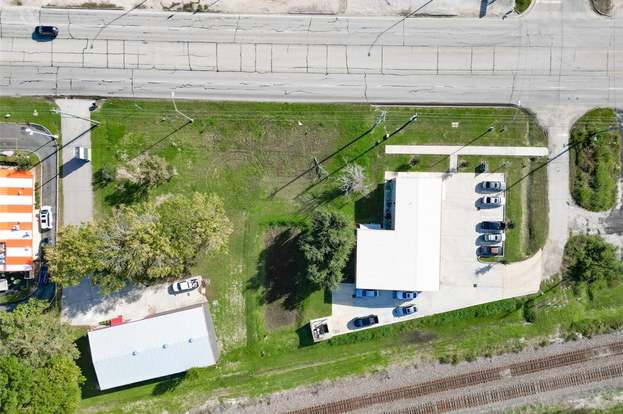An overhead satellite image captures a desolate, rural town featuring both residential and commercial buildings. The scene includes a large, worn-down road with minimal traffic—only a single vehicle is visible—paralleling a set of commercial buildings. In front of these buildings, the road's deteriorated state is evident. The landscape around the area is predominantly green, adding to the rural atmosphere.

The buildings are arranged linearly from left to right. The first building has a red and white striped roof with a circular driveway. Behind and slightly right of this structure is a gray warehouse-like building, followed by a larger, irregularly shaped building with a sloped white or light gray roof. This largest building, notable for having the most vehicles parked outside, features an extension at the rear and two separate driveways connecting it to the main road. All three buildings have vehicles parked in front of them and are serviced by overhead power lines.

In the bottom right of the image, there is a double set of railroad tracks running diagonally, with one incoming and one outgoing. No trains are present at the moment. The combination of industrial, commercial, and residential elements set against the backdrop of an underpopulated, rural environment paints a picture of a sparsely inhabited town.